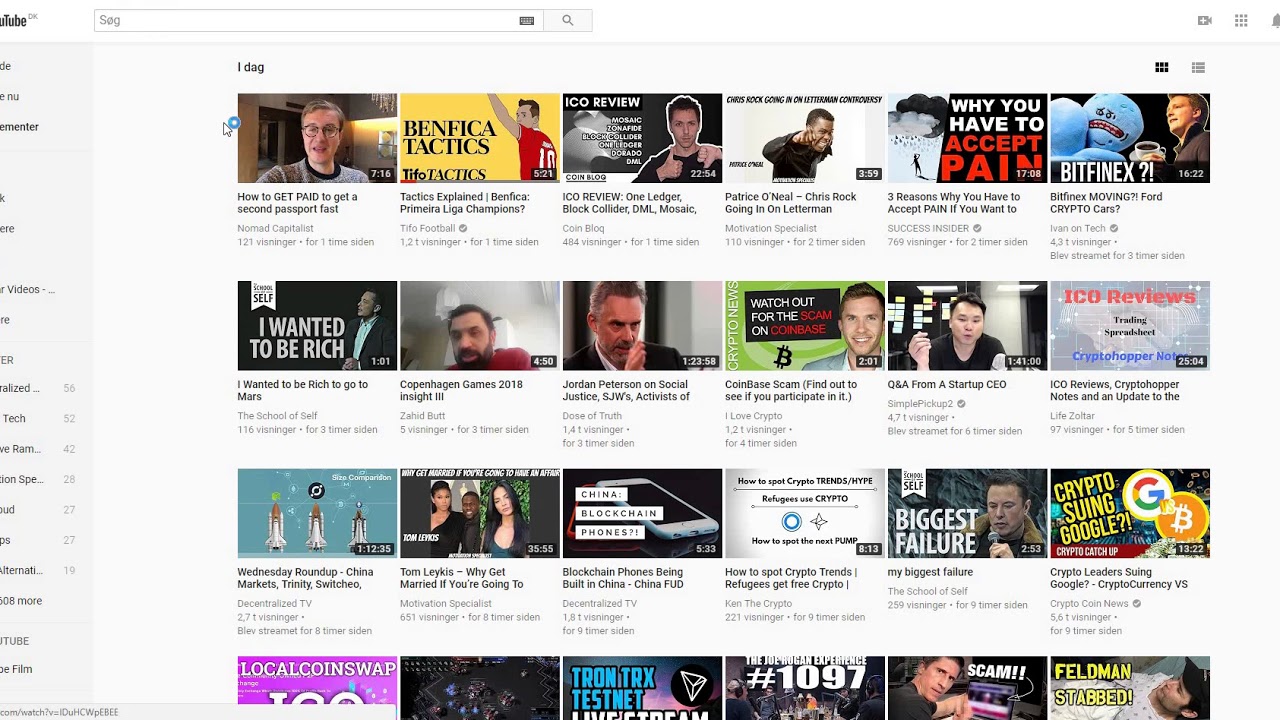The image is a screenshot taken vertically from a computer screen or smartphone, depicting a partially captured view of YouTube. In the upper left-hand corner, the YouTube logo is visible but partially cut off, showing only part of the "U" and the full word "Tube." Below the logo, there is a long, slender search bar with the text "SOG" typed in it, accompanied by a magnifying glass icon for search. 

On the left side of the screen, a gray sidebar displays partially visible and cut-off navigational options. The background becomes lighter as it stretches to the right side of the image. At the top center-right of the screen, the word "iDog" is written in black. Below "iDog," there is a grid of YouTube video thumbnails, organized in a 6-column layout. However, only 4 rows are visible, with the bottom row partially cut off.

Each video thumbnail includes a short description underneath. The first video reads, "How to Get Paid to Get a Second Passport Fast," authored by "Named Capitalist," with a timestamp of "121:04," and labeled as "one time cited." In the upper corners of the image, additional icons are present, providing more options but not fully discernible due to the partial capture.